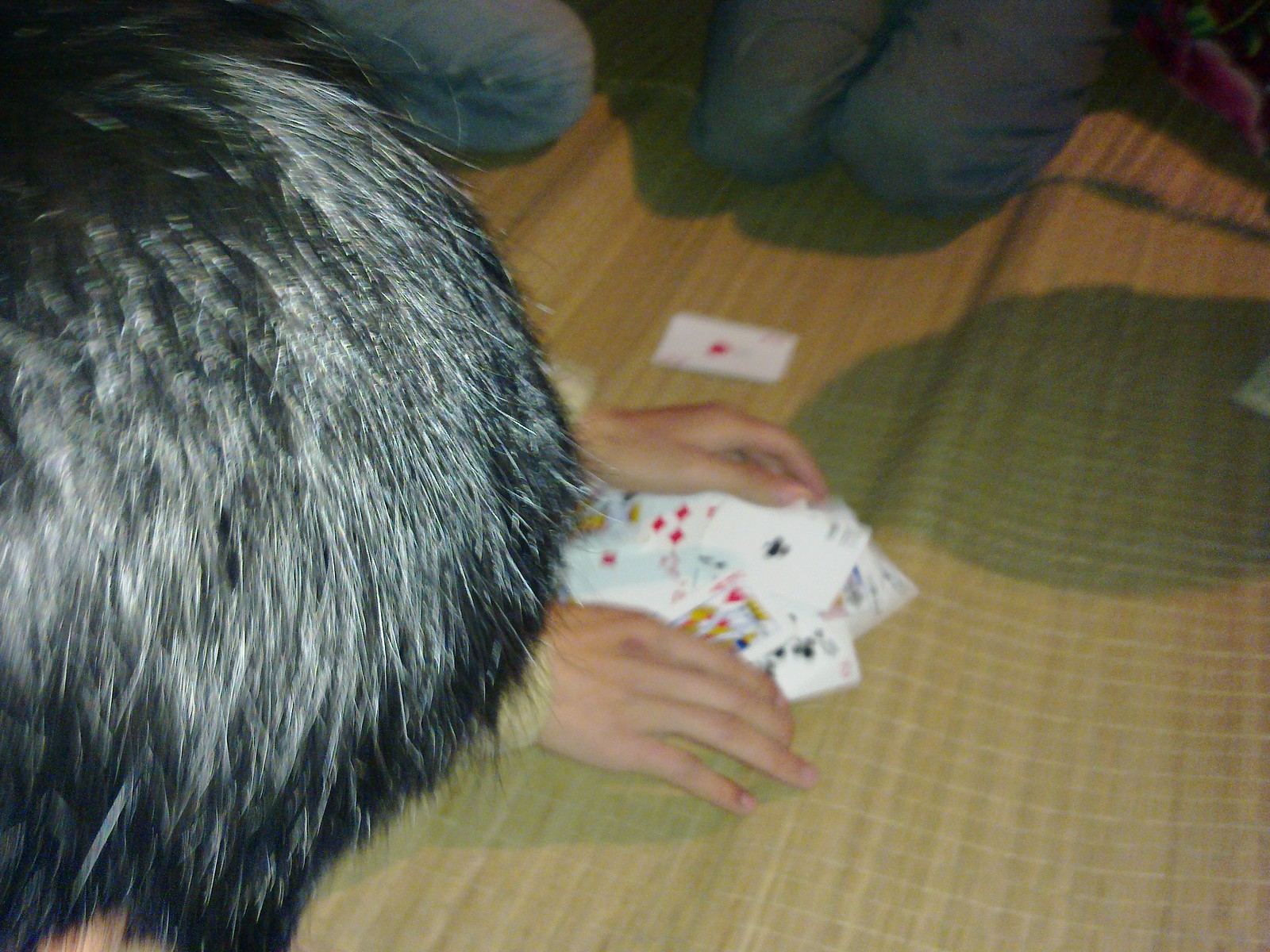In this photograph, a group of people are engrossed in a game of cards, seated on what appears to be a bamboo mat spread out on the floor. The mat serves as a soft and natural floor covering, creating a casual and relaxed atmosphere. In the center of the mat, two hands are seen reaching towards a scattered pile of playing cards, which, though somewhat blurry, reveal various suits and face cards. Just above the cards, a pair of knees are visible, indicating that at least one person is kneeling as they play. Closest to the camera is the back of someone's head, featuring thick, short, and spiky black hair. The image captures a candid and intimate moment, without any accompanying text.